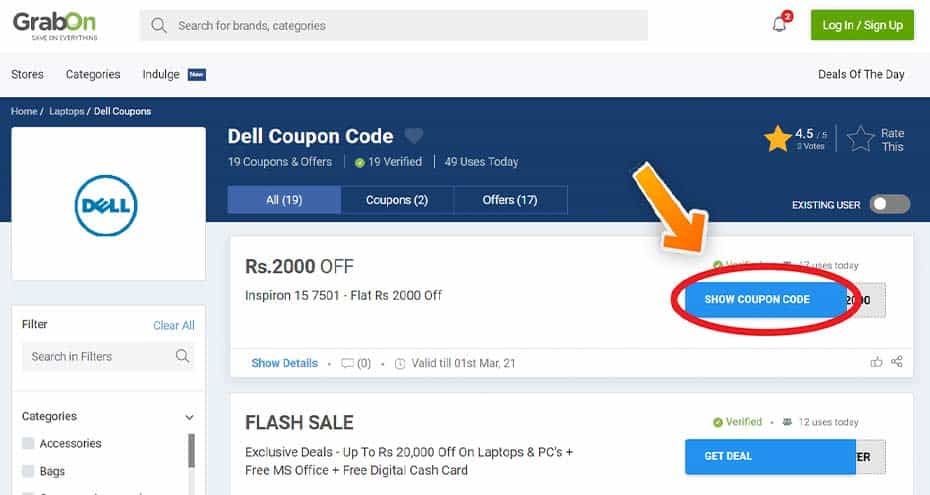The image displays a web page named "GrabOn," as indicated in the upper left-hand corner. The name is stylized with "Grab" in black and "On" in green, all written as one word. At the top of the page, there is a search bar and navigation options labeled "Stores," "Categories," and "Indulge." Additionally, there is a Dell emblem featuring a teal circle with the word "Dell" inscribed inside.

In the top right-hand corner, there is a green login section labeled "Login/Sign Up," accompanied by a notification bell displaying either the number 2 or 3, indicating unread messages. 

A prominent feature highlighted on this page is a Dell coupon code section. An orange arrow is pointed downward towards a blue rectangular button labeled "Show Coupon Code," which is circled by a red oval.